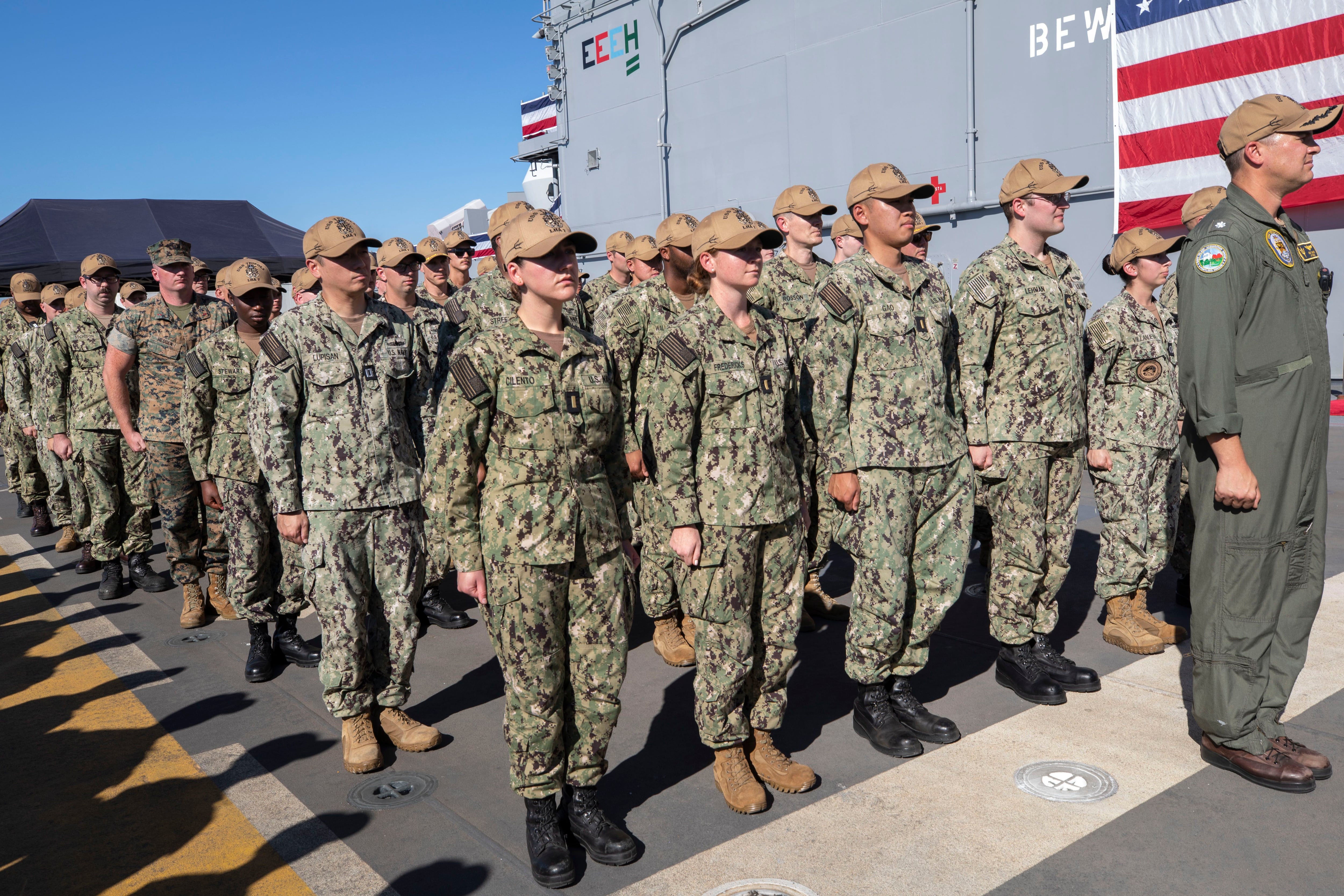In this horizontal landscape image, a group of predominantly white male and female army soldiers stands outdoors during the day, arranged in neat rows of five at attention. They are all dressed in green and brown camouflage military fatigues with tan baseball caps, and are wearing either black or brown boots. Among them, positioned towards the right edge of the image, is a leader distinguished by an olive jumpsuit and brown leather shoes, also sporting a tan baseball cap. Above this leader's head, part of an American flag with visible red and white stripes and a star on a blue background can be seen. The assembled soldiers cast distinct shadows towards the lower left corner of the image, and in the background on the upper right, part of a gray wall with the white text "B-E-W" and "E-E-E-H" is visible against a blue sky.